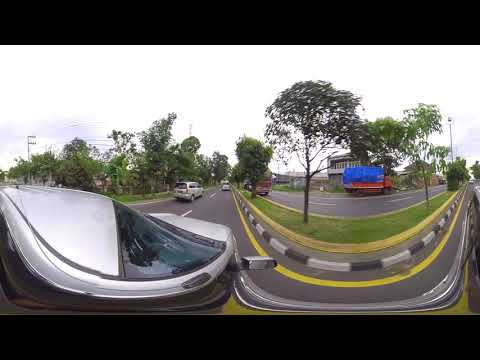The image captures a dynamic scene from a moving vehicle, potentially a car, taken with a fisheye lens that creates a noticeable distortion. The photo showcases a busy street with multiple vehicles ahead, including a warped car directly in front on the left side. The scene is set on the right-hand side of the road, featuring a painted curb with alternating black and white stripes and a yellow line running alongside it. Across the median with trees, there is a truck covered with a blue tarp, possibly transporting bales of hay. The surroundings include several buildings visible in the distance, along with a clear sky adorned with some clouds. The varied colors in the image span from the natural hues of the surroundings to the vibrant shades of the vehicles, emphasizing the outdoor setting in the middle of the day.